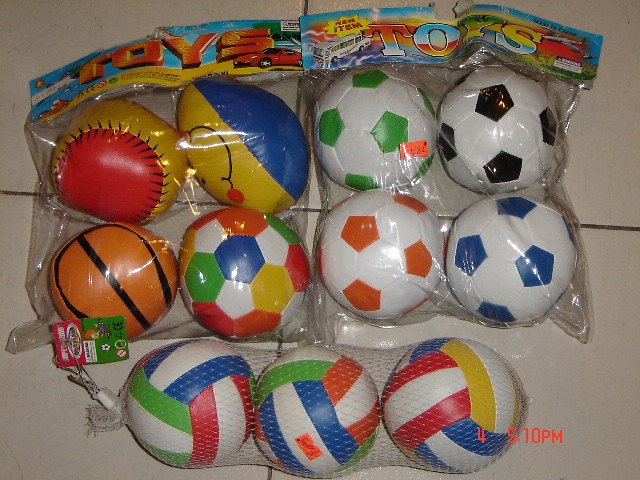The image shows three distinct packages of toy balls displayed on a white tile surface. Positioned in the top left is a plastic bag with a cardboard label that reads "Toys" in large orange letters. It contains four balls: a baseball colored gold and red, a blue and yellow football featuring a big smiley face, an orange basketball with black stripes, and a multicolored soccer ball with patches of green, white, blue, and orange. Adjacent to this, the top right plastic package, similarly labeled "Toys" and marked with an orange price sticker, also contains four different colored soccer balls—primarily white with accent colors of green, black, orange, and blue. Below these, there's a long, tube-shaped mesh bag tied at the top. This bag holds three striped balls resembling volleyballs or water polo balls, featuring color combinations of blue and white, green and white, and red and white. The distinctive packaging and the variety of ball types are underscored by the time stamp "4 5:10 PM" in the lower right corner of the image.